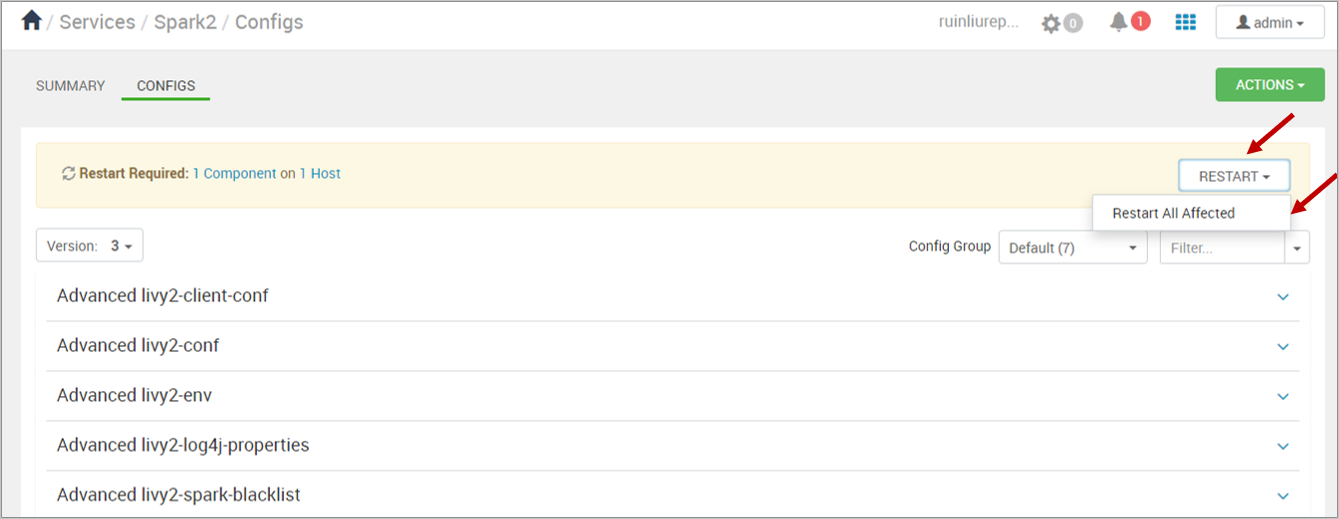**Caption:**

The image is a detailed screenshot of a configuration window. The interface has a predominantly white background with black text. At the top left corner, a home icon is displayed, followed by the menu labels "Services," "Spark 2," and "Configs" in gray text. On the top right, there is a username, "RuinLerip," in gray, accompanied by a gray settings gear icon with a number zero next to it. Adjacent to these, a gray notification bell icon shows a red number one alert, a blue 3x3 grid menu icon, and a user icon with a drop-down menu labeled "Admin."

Below the top bar, a gray background section is divided into "Summary" and "Configs," with "Configs" highlighted by a green underline, indicating it is the selected tab. On the right, there is a prominent green drop-down button labeled "Actions" in white text. Under this header, a noticeable pink bar stretches across the screen displaying "Restart Required: one component on one host." Beneath this alert, various configuration drop-down options are listed, such as "Advanced LIV2 Client Config," "Advanced LIV2 Config," "Advanced LIV2 Env," and "Advanced Load Properties," among others.